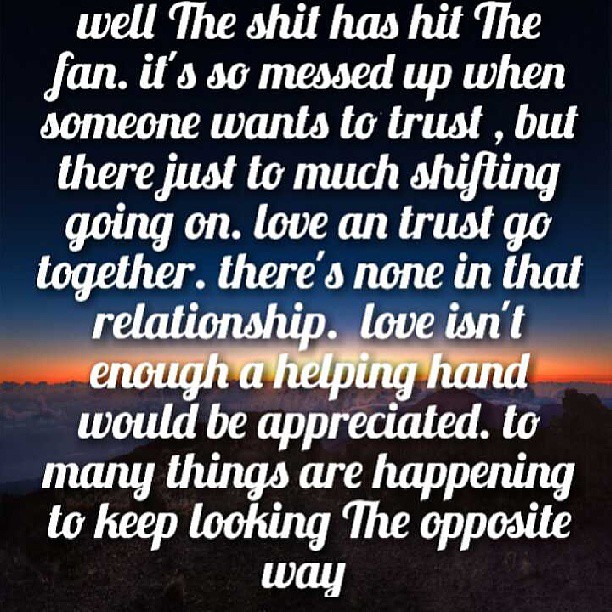This color photograph, often referred to as a meme, features a poorly written text post overlaid on a sunset background. The image displays a dark blue sky transitioning into a small sliver of orange, indicating the setting sun. The landscape appears to be a mountain range, but the image is largely obscured by the text, making it difficult to discern the exact scenery. The text is written in thick, white cursive script and reads: "Well, the shit has hit the fan. It's so messed up when someone wants to trust, but there's just too much shifting going on. Love and trust go together. There's none in that relationship. Love isn't enough. A helping hand would be appreciated. Too many things are happening to keep looking the opposite way." The caption is riddled with grammatical errors, including incorrect usage of "TO" instead of "TOO," inconsistent capitalization, and misspelled words such as "A-N" instead of "AND."